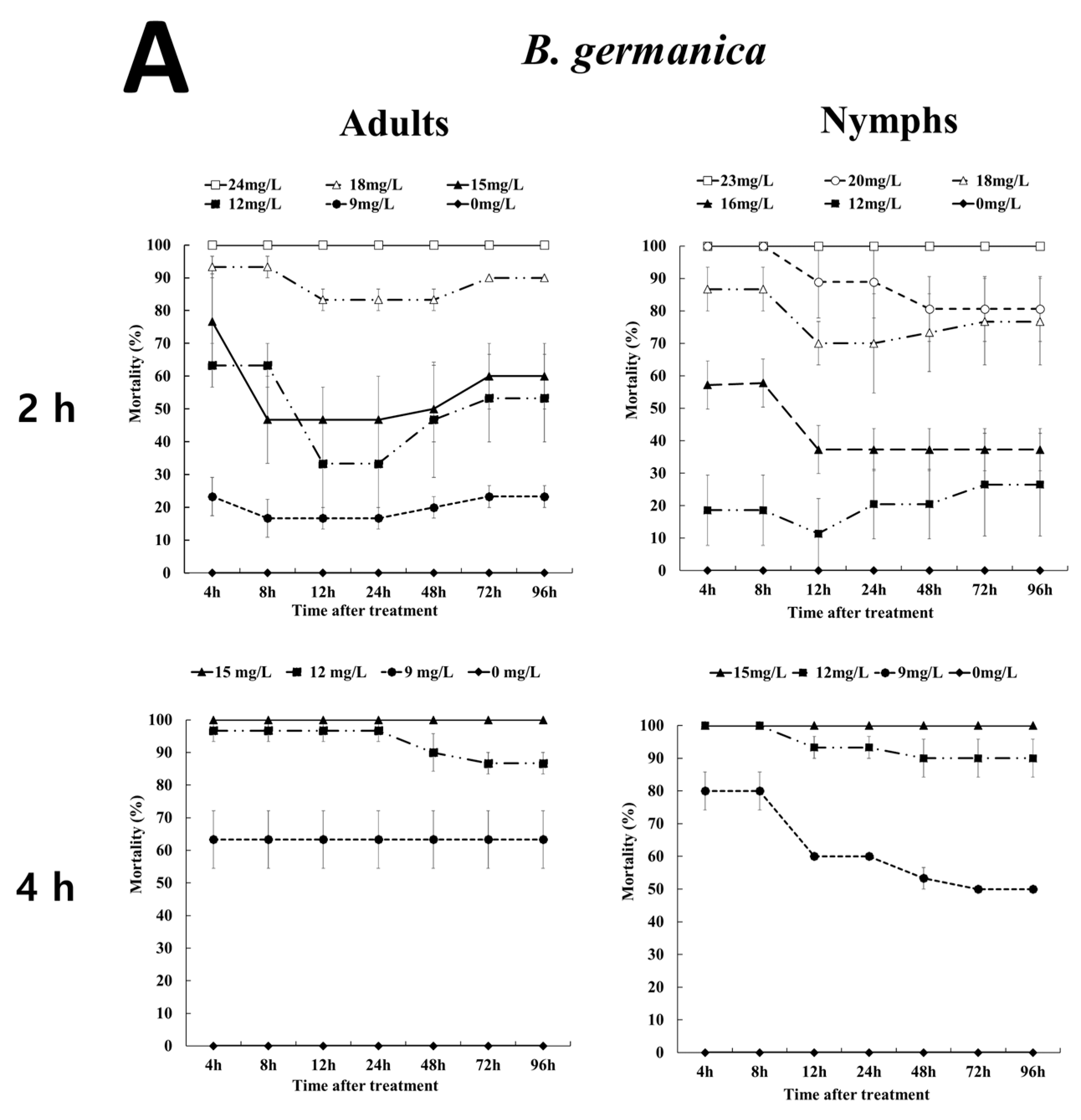The image features four line graphs against a white background, grouped under the heading "B. Germanica" in the top center. The graphs are categorized into two main groups: "Adults" on the left and "Nymphs" on the right. A prominent letter "A" appears in the upper left corner of the image.

For each category, there are two graphs: one in the top row labeled "2 hours" and one in the bottom row labeled "4 hours." Each graph shares the same axes: the x-axis represents time after treatment, ranging from 4 to 96 hours, and the y-axis indicates mortality percentage, from 0% to 100%.

In the "Adults" section:

- **2 Hours (Top Left Graph):** Features 5-6 lines with different markers showing varying MGL (possibly microgram levels): white square (24 MGL), white triangle (18 MGL), black triangle (15 MGL), black square (12 MGL), black circle (9 MGL), and small black diamond (0 MGL).
  
- **4 Hours (Bottom Left Graph):** Displays 3-4 lines with fewer markers: triangle (15 MGL), square (12 MGL), circle (9 MGL), and small diamond (0 MGL).

In the "Nymphs" section:

- **2 Hours (Top Right Graph):** Includes 5-6 lines representing different MGL levels: white square (23 MGL), white triangle (18 MGL), black triangle (16 MGL), white circle (20 MGL), black square (12 MGL), and black diamond (0 MGL).
  
- **4 Hours (Bottom Right Graph):** Contains 4 lines marked with: black square (12 MGL), black star (15 MGL), black square and circle (9 MGL), and black diamond (0 MGL).

Each graph uses solid and dashed lines with distinct markers to differentiate the treatment levels over time, illustrating mortality percentages in a non-linear fashion with various peaks and troughs across the recorded time points.